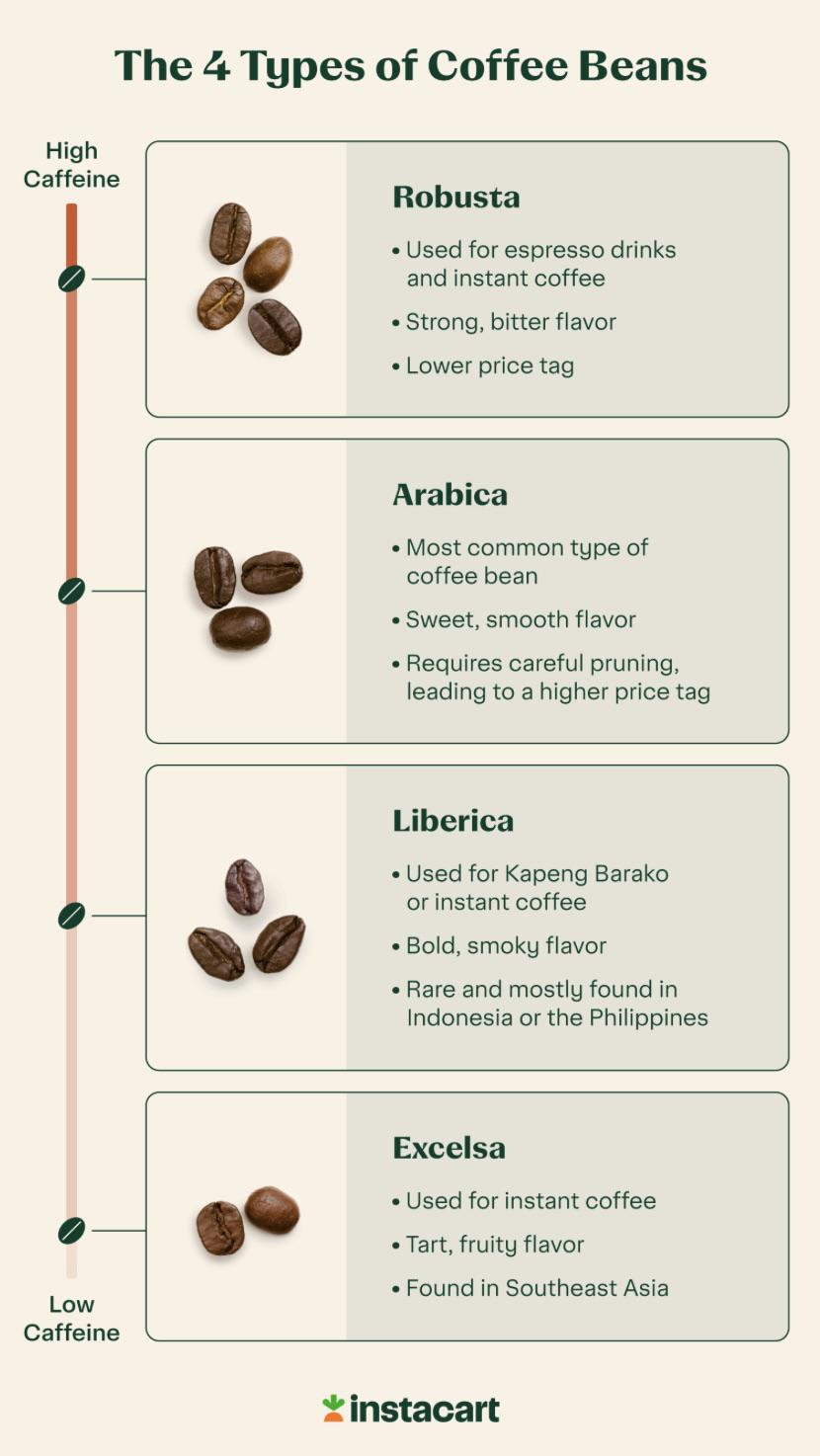This detailed infographic showcases the four types of coffee beans on a rectangular, light brownish-pink background. The chart, approximately five inches high and three inches wide, is topped with a bold green heading: "The Four Types of Coffee Beans."

To the left of the chart, a vertical stripe transitions from dark orange at the top to pale at the bottom, labeled "High Caffeine" above and "Low Caffeine" below. Alongside this gradient, four green coffee bean icons point to four rectangular sections that include detailed descriptions and images of each coffee bean type.

1. **Robusta**: 
   - Image: Four dark brown roasted coffee beans
   - Usage: Espresso drinks and instant coffee
   - Flavor: Strong, bitter
   - Price: Lower price tag
   - Caffeine Level: Highest

2. **Arabica**: 
   - Image: Three dark brown roasted coffee beans
   - Usage: Most common type of coffee bean
   - Flavor: Sweet, smooth
   - Price: Higher due to careful pruning
   - Caffeine Level: Moderate
   
3. **Liberica**: 
   - Image: Three slightly shriveled, dark brown coffee beans
   - Usage: Kapang Barako or instant coffee
   - Flavor: Bold, smoky
   - Rarity: Rare, mostly found in Indonesia or the Philippines
   - Caffeine Level: Moderate
   
4. **Excelsa**:
   - Image: One split roasted coffee bean, showing two halves
   - Usage: Instant coffee
   - Flavor: Tart, fruity
   - Location: Found in Southeast Asia
   - Caffeine Level: Lowest

Below the descriptive sections is the Instacart logo, a green stem and orange carrot symbolizing the brand. The vertical stripe on the left effectively communicates the caffeine content, transitioning from high at the top with Robusta to low at the bottom with Excelsa, offering a comprehensive, visual representation of the caffeine levels amongst the four coffee bean types.